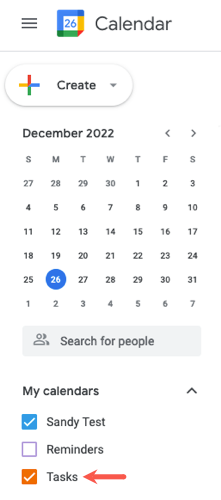The image displays a calendar interface on a cell phone screen. In the top left corner is a menu tab icon, followed by a square icon with various colored squares centered within it and labeled with the number "26." To the right is the text "Calendar." Below this text, there is a thin horizontal gray line. Underneath the line is a large white oval button featuring a plus sign surrounded by quadrants colored green (bottom), yellow (left), red (top), and either orange or blue (right), which is labeled "Create" with a downward arrow beside it.

The main portion of the screen showcases the monthly calendar for December 2022, organized from Sunday to Saturday. The calendar starts from Sunday, November 27th, and ends at Saturday, January 7th. The date 26th, which falls on a Monday, is highlighted with a blue circle, indicating it is selected.

Below the calendar, there's a light gray search bar displaying the prompt "Search for people." Beneath this search bar is a section titled "My Calendars," listing three calendar items: 

1. A blue square with a check mark labeled "Sandy Tests."
2. An unchecked option labeled "Reminders."
3. An orange square with a check mark labeled "Tasks" that includes a red arrow pointing to it.